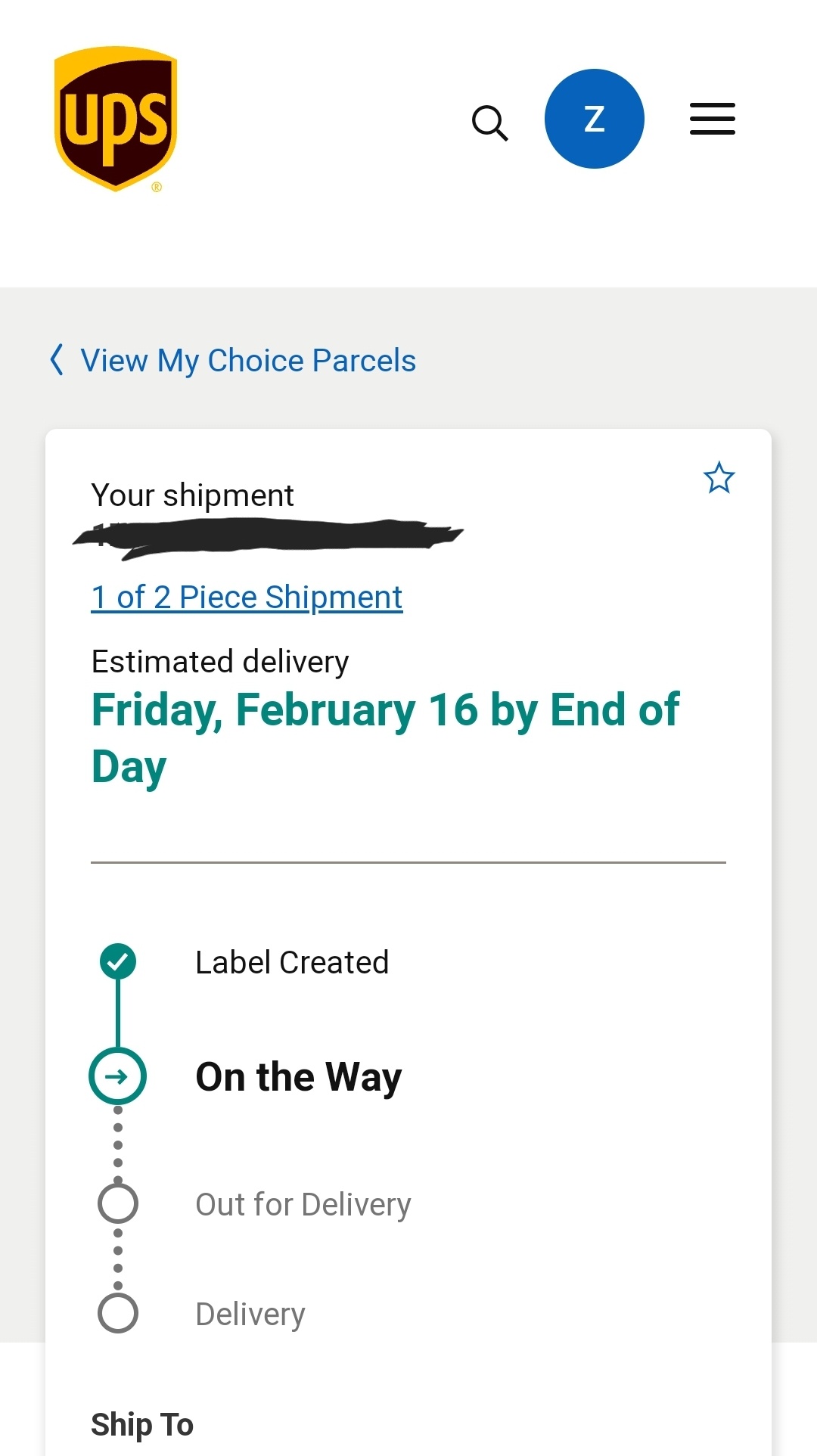In the top left corner of the image, there is a UPS logo, shaped like a shield. The logo has a predominantly dark brown background, but at the top, there's a slanting section that ascends to the right and transforms into a yellow background, which borders the entire logo. The letters "UPS" are displayed in yellow.

To the right of the logo, there is a magnifying glass tilted to the left. Adjacent to the magnifying glass is a solid dark blue circle with a white capital "Z" in its center. To the right of the circle, there are three black horizontal lines indicating a drop-down menu.

Below this area, there is a rectangular section with a light gray border. The top part of this border is significantly thicker and displays the text "View My Choice Parcels" in dark blue, accompanied by an arrowhead pointing to the left.

The main content of the section is a white rectangle with the text "Your Shipment" in black. Under this text, the content is obscured by black strike-through lines. Beneath the blacked-out section, there is a bluish-green band with the text "1 of 2 Piece Shipment" in white.

Further down, in black text, it reads "Estimated Delivery," followed by bold teal lettering stating "Friday, February 16 by End of Day," with the "E" in "End" and the "D" in "Day" capitalized. A gray line serves as a border illustrating the progress of the delivery.

The delivery progress starts with "Label Created," marked by a small filled-in teal circle containing a white checkmark. A solid teal line connects this to a larger teal-bordered circle with an arrow pointing right, labeled in bold as "On the Way," indicating the current step. Gray dots extend from there to a gray outline circle labeled "Out for Delivery," followed by more gray dots leading to another gray circle labeled "Delivery."